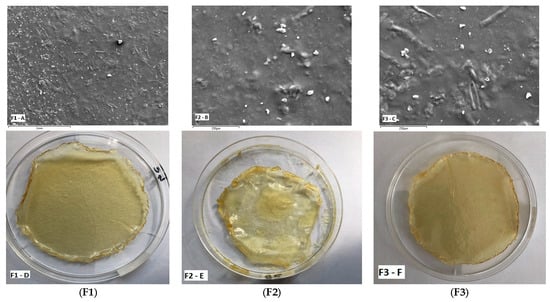The image depicts a scientific experiment displayed in six pictures arranged in two rows and three columns. The top row features three images showing a rough, gray surface that resembles the moon, dotted with white specks. The bottom row shows three clear circular petri dishes, each containing a round yellow layer, serving as a frame. These dishes are placed on a white table. The columns are labeled F1, F2, and F3 respectively. Based on the arrangement and the labels, it appears that each column corresponds to a specific sample at different stages or conditions, with microscopic images above and macroscopic images below. The labels and content suggest that the images are recording changes or consistencies in the samples, with the middle sample showing a higher concentration of white specks compared to the first and third samples.